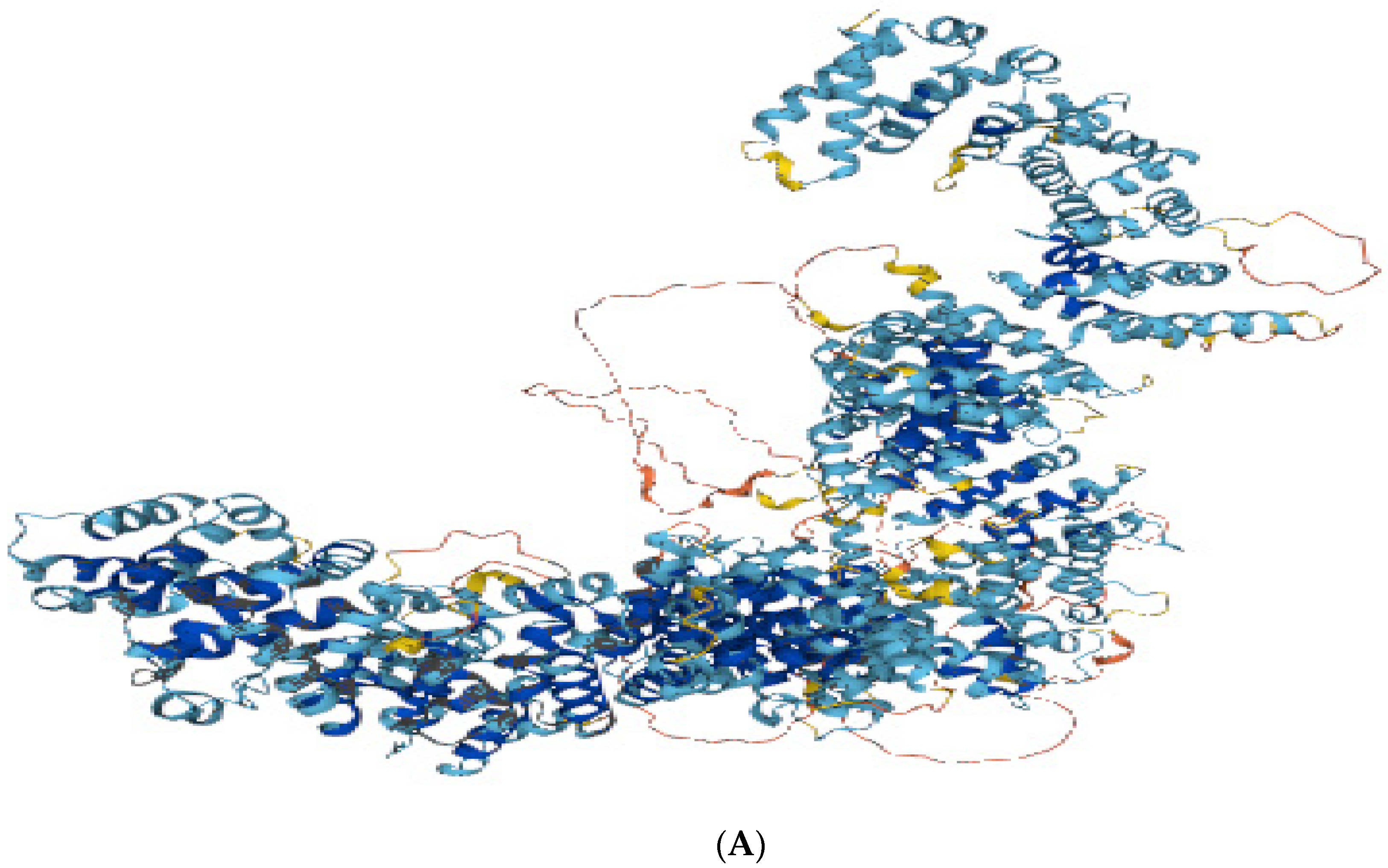The image features a complex, intertwined bundle of spiral ribbons predominantly in shades of dark blue and light blue, with accents of green, orange, and yellow, as well as sporadic red strings interwoven throughout the structure. The ribbons resemble curly strands, possibly indicative of a microscopic view of a virus's DNA structure. The background is white, providing a stark contrast that emphasizes the vivid colors and intricate details of the ribbons. The entire composition extends from the top right down to the bottom left of the image, where the letter "A" is displayed in black font within parentheses, anchoring the visual. The design's appearance, with its spiraled and wiry textures, gives an impression of both scientific illustration and abstract art.